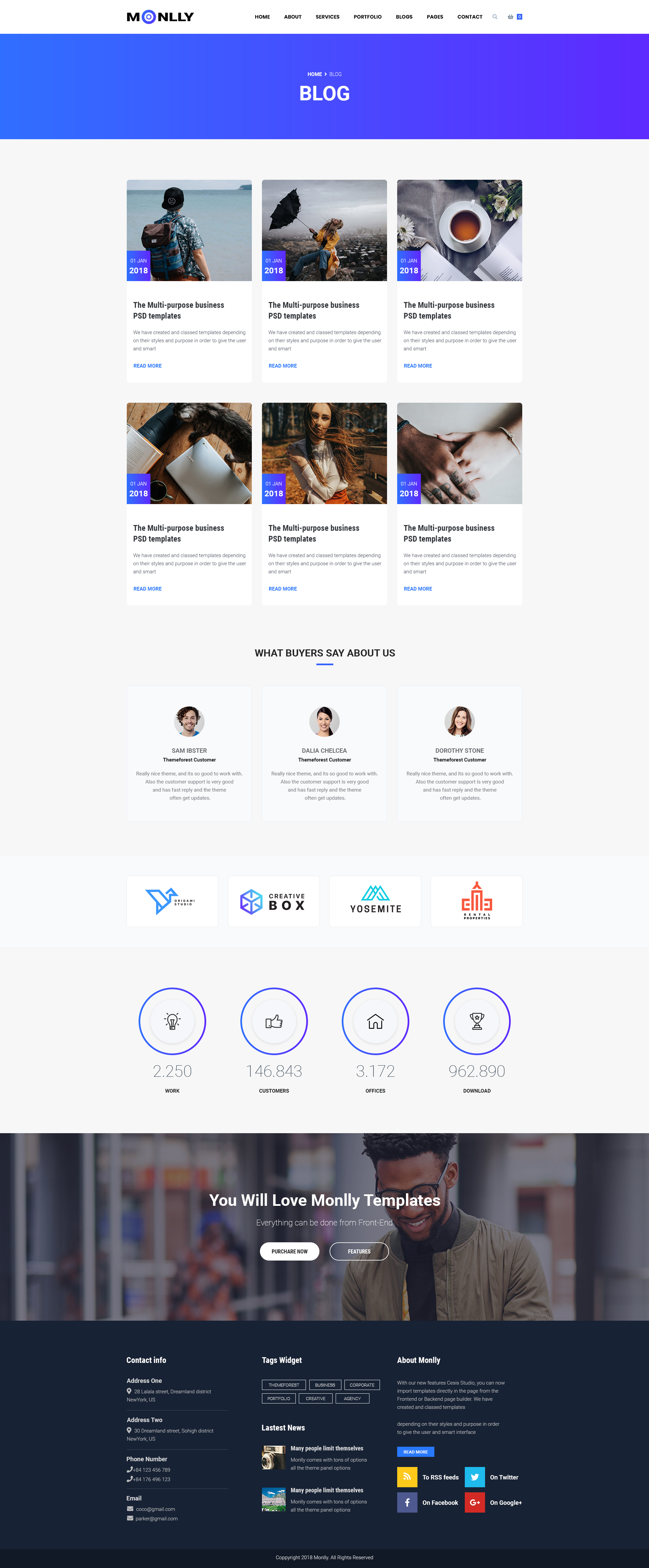The image is a screenshot of a webpage that presents several quality issues, such as being very small and having mediocre resolution, making most of the text unreadable. Starting from the top, there's a blue border beneath which lies a navigational menu on a white background; however, the text on this menu is too small and blurry to decipher. The company name appears to be "MONILLY" rendered in a bold black font except for a blue 'O'. 

Below this, the word "BLOG" is prominently displayed in a large, readable white font on the blue border. The main content of the page features a white background with six photos arranged in a 3x2 grid. Each photo has a caption underneath, which is not readable. The top right image depicts a table with a white bowl of soup, while the bottom center image showcases a white woman with reddish-brown hair.

Further down, a headline reads, "What Buyers Say About Us," indicating the presence of testimonials which are accompanied by three tiny headshots. The headshots include two white women on the left and right, and a white man in the center. 

At the bottom of the webpage, logos of various companies such as Box and Yosemite are displayed, although two others are not discernable. The footer area features a partially visible image of a black man wearing dark glasses and an army-green jacket. Accompanying this image, a headline states, "You Will Love Monili Templates." The footer itself has a dark bluish-gray background with unreadable text but includes recognizable icons for Facebook, Twitter, and a couple of others which are yellow and red.